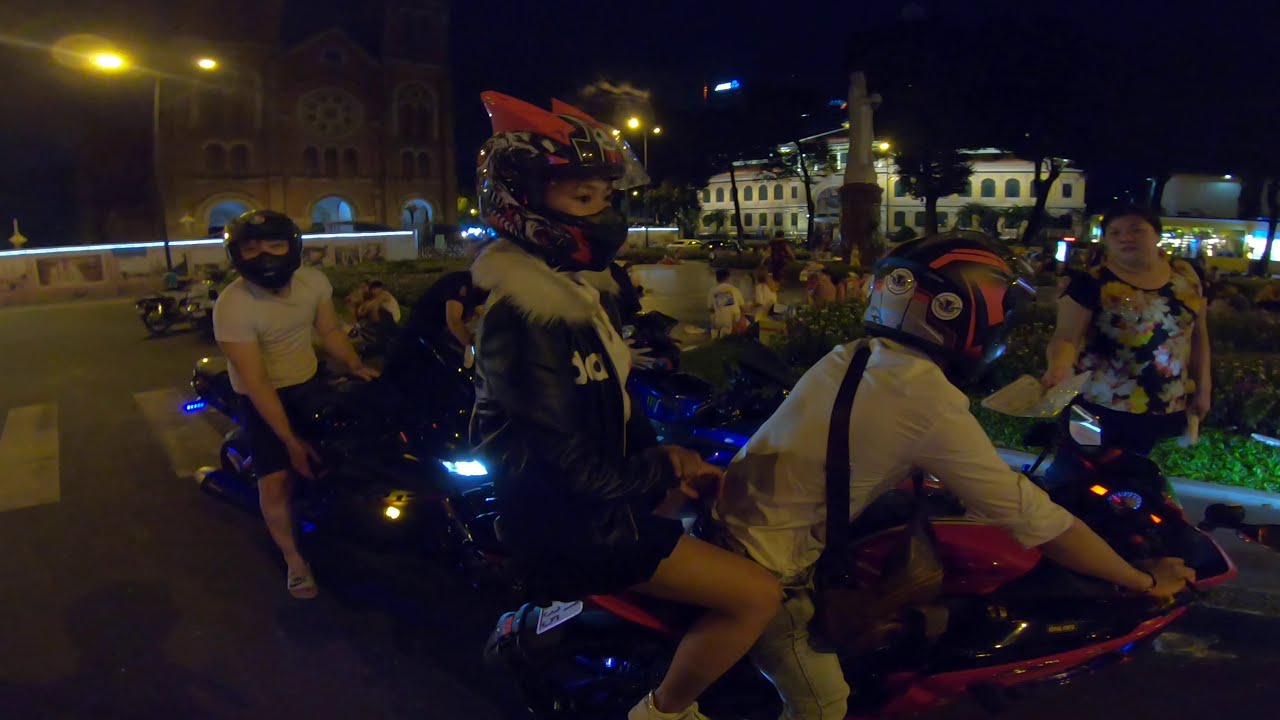In this nighttime outdoor scene, a bustling city center, likely Ho Chi Minh City, comes to life with a group of motorcycle riders. At the forefront, a prominent red and black motorcycle is navigated by a man in a white button-down shirt, with a woman in a black jacket with a fuzzy collar and a helmet adorned with red fins sitting behind him. Nearby, a woman in a flowered shirt stands by, handing a piece of paper to another rider. 

Around them, several other motorcycles, predominantly in darker black colors, are visible, driven by helmeted riders as well. The background showcases grand, older buildings illuminated against the night sky, suggesting an ambience of historical richness. Additionally, there’s a well-lit, manicured garden area where people are seated, possibly socializing around a majestic statue that stands at its center, contributing to the locale's charm and cultural intrigue.